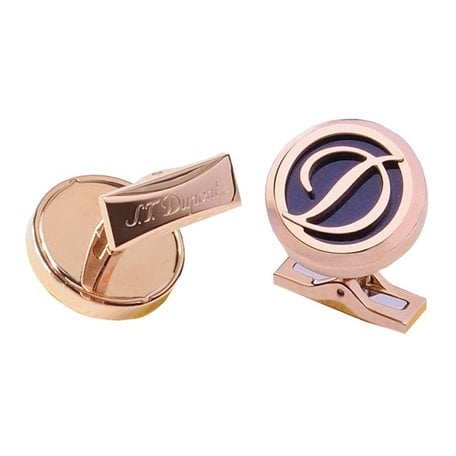This photograph showcases a pair of elegant, rose gold-colored cufflinks set against a white background. Each cufflink features a circular face and a rectangular fastener, embodying a classical and stylish design that suggests they could be quite expensive. The cufflink on the right displays its circular face prominently, adorned with a large, italicized letter 'D' in rose gold against a deep purple background. In contrast, the cufflink on the left reveals the underside of the rectangular fastening mechanism, where the brand name "St. DuPont" is scripted in cursive, albeit slightly reflective and challenging to read due to its shiny finish. The picture smartly positions the cufflinks to exhibit both their decorative and functional aspects, underlining their sophisticated appeal and meticulous craftsmanship.